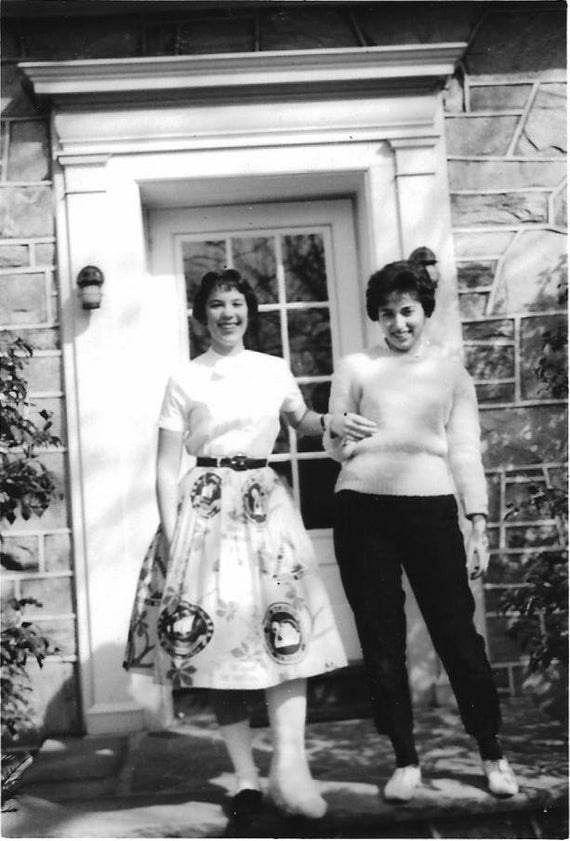The black and white photograph captures a poignant moment between a younger girl and an older woman, both smiling warmly as they stand together in front of a doorway. The doorway is distinctive with its ornate white frame that includes crown molding and raised white pillars. Attached to this frame are two lights, one on each side. The door itself is white, featuring a large rectangular window with several small panes divided by white lines. Behind them, the house appears to be made of brick, or possibly stone, which adds a textured backdrop to the scene.

The younger girl, standing on the left, has short black hair and is dressed in a white shirt paired with a patterned white skirt adorned with floral designs and small black circled white ducks. She wears white socks and black shoes, but notably, her left leg is in a cast. The older woman stands to the right, holding the girl's left arm supportively. She has curly short black hair and wears a white sweater, black pants, and white shoes. The clear and well-lit setting emphasizes their joyful expressions and the intimate bond they share.